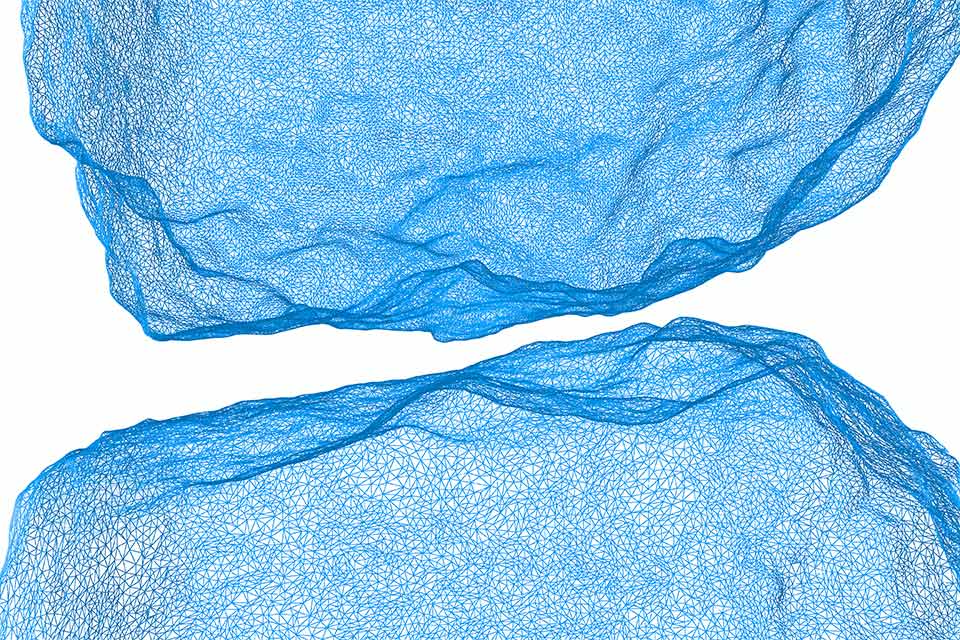The image features two irregular, semi-circular shapes positioned on a white background, with one shape extending from the top of the picture into the middle and the other from the bottom. Rendered entirely in blue ink, these shapes resemble abstract, computer-generated rock forms with rough, crinkled edges that give them an aged and pitted appearance. Both shapes fill nearly the entire width of the image and exhibit a textured, almost web-like geometric pattern composed of thin blue lines. Despite their irregular forms, they mirror each other in appearance, creating a symmetry that is both distinct and cohesive. The negative space of white between and around them further accentuates their uniqueness and draws attention to their intricate details.